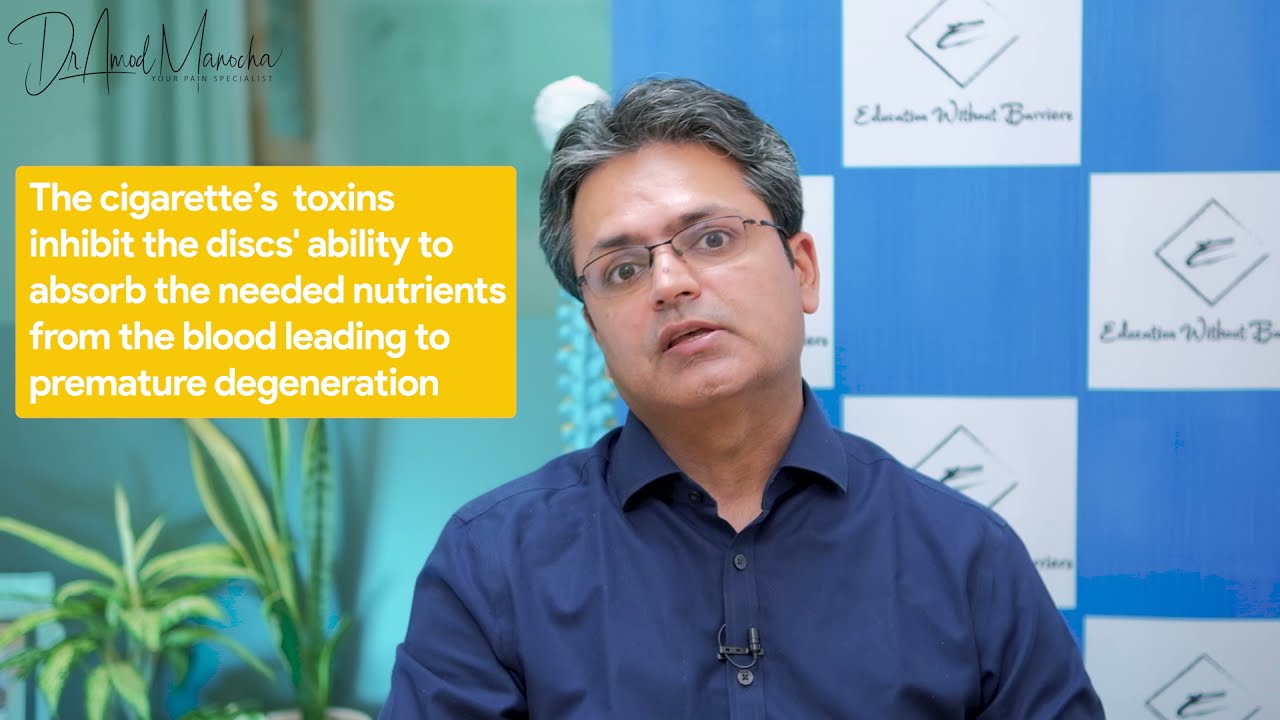This image captures a screenshot from a quit smoking seminar, featuring a middle-aged man of possibly Southeast Asian or Indian descent, who appears to be Dr. Arnaud Manocha. He is around 45 years old with speckled black and gray hair parted down the center, and rimless glasses. His head is tilted to the top left, and his mouth is slightly open, showing the edges of his teeth, as if he's in the middle of speaking. He wears a navy blue button-down collared shirt with a small microphone clipped between the first and second buttons. To the left of the man is a yellow text box with white text that reads, "The cigarette's toxins inhibit the disc's ability to absorb the needed nutrients from the blood leading to premature degeneration," spread over five lines. In the background, there is a blue and white checkerboard pattern featuring white squares with a cursive logo resembling a pistol with a tail and some illegible text below. To the bottom left of the man is a cluster of green plants. The upper left corner of the text box showcases a stylized signature that likely reads "Dr. Ahmad Minocha," with the subtitle "your pain specialist" in all caps. The setting appears professional, akin to a video presentation or seminar.